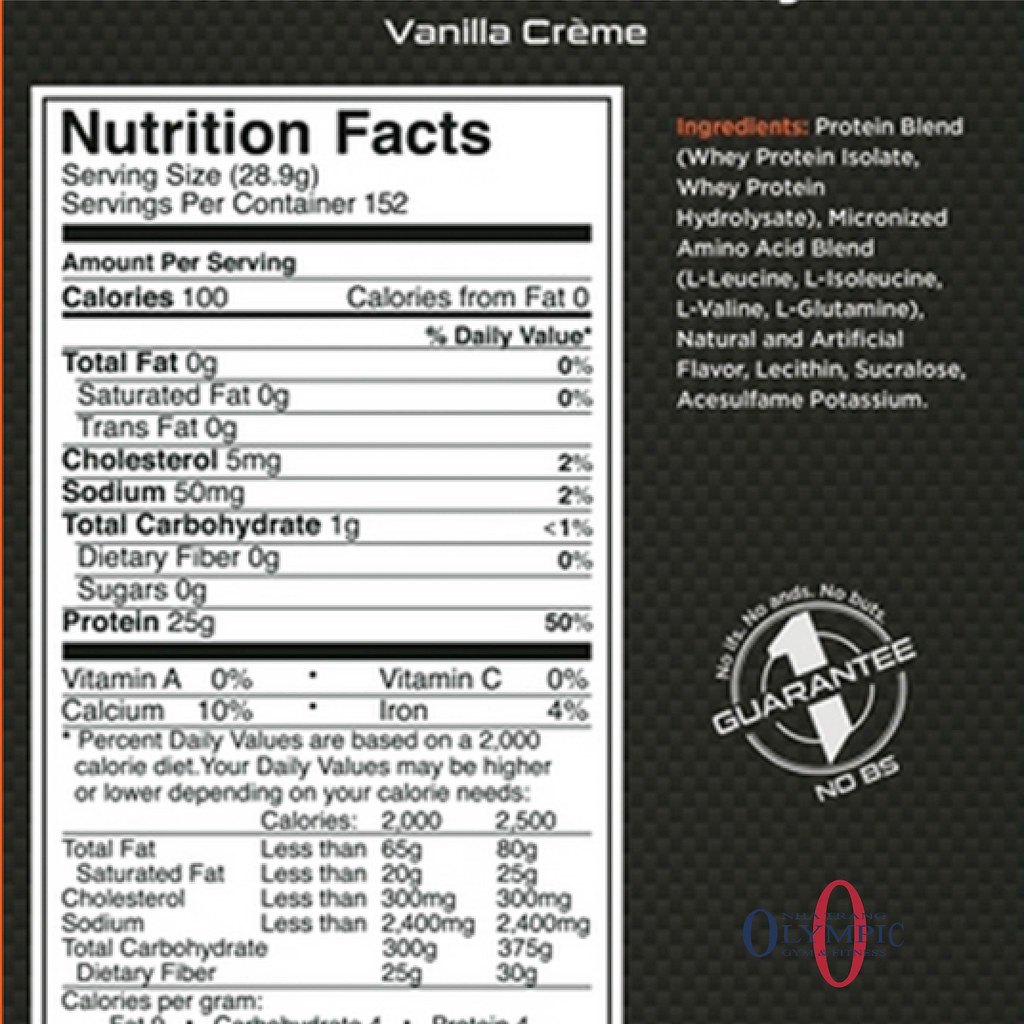This is an image of a label for a protein drink with a dark gray, textured background reminiscent of a shelf liner. At the top, in white text, it reads "Vanilla Crème." On the left side of the label, a large white rectangle contains the nutrition facts, detailed in black font. This section lists vital information such as servings per container (152), calories per serving (100), and an array of nutritional values including fat, saturated fat, trans fat, cholesterol, sodium, carbohydrates, sugars, and notably, 25 grams of protein per serving. Below these are listed the specific vitamins and minerals the drink contains.

The right side of the label features the ingredients section written in white text on a transparent background revealing a pattern of 3D triangles. The word "ingredients" is highlighted in red. This section identifies the presence of whey protein isolate, other proteins, amino acids, and various vitamins. 

Prominently stamped at the bottom of the ingredients list is the guarantee that reads, "No ifs, no ands, no buts. Number one guarantee, no BS," accompanied by a large red zero or "O." Below this guarantee, there is an additional symbol that blends blue and red colors, although the details of this symbol are not entirely clear.